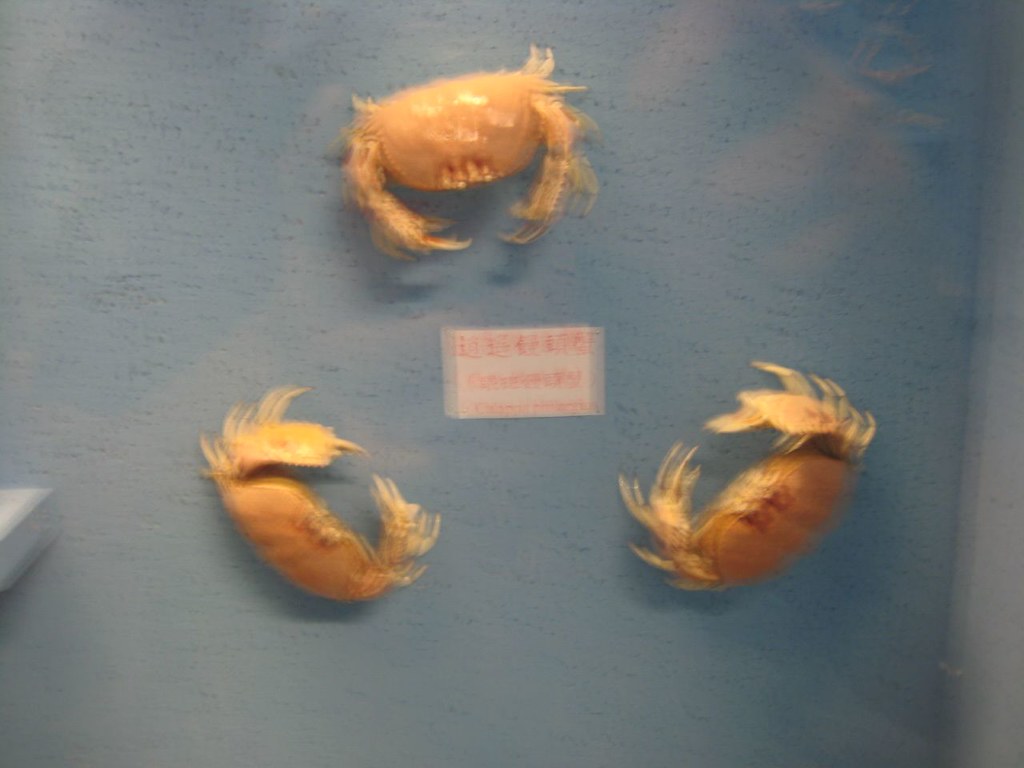This blurry photograph captures three pale reddish-tan crabs arranged in a triangular formation on a blue and gray background, possibly a floor-like carpeting or cloth. The crabs, with their claws extended and eyes protruding from their oval-shaped bodies, appear to be interacting or potentially confronting each other. At the center of the triangle, there is an unreadable piece of paper with red lettering. Additionally, there is an indistinct box-like object toward the left-hand side of the image. The overall composition suggests a dynamic, albeit unclear, scene.